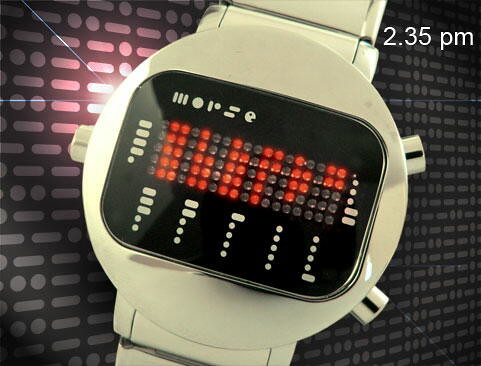The image features a futuristic, possibly vintage, digital watch with a distinctive and intricate screen. The watch itself has a sleek silver exterior and an unconventional face that doesn’t display numbers in the traditional sense. Instead, the screen is filled with a grid made up of various Braille-like dots arranged in a four by two layout. These dots are either gray or illuminated in red, suggesting some form of tracking or rendering process. The outer frame of the watch is white, providing a striking contrast to its detailed, high-tech interior. In the top right corner of the image, a watermark displays the time "2:35 p.m." against a black background. The layout also includes pink and white ovals and circles towards the left side, contributing to a stylish and modern advertisement aesthetic. The overall lighting is bright, particularly from the left side, emphasizing the watch's glossy finish and detailed elements.